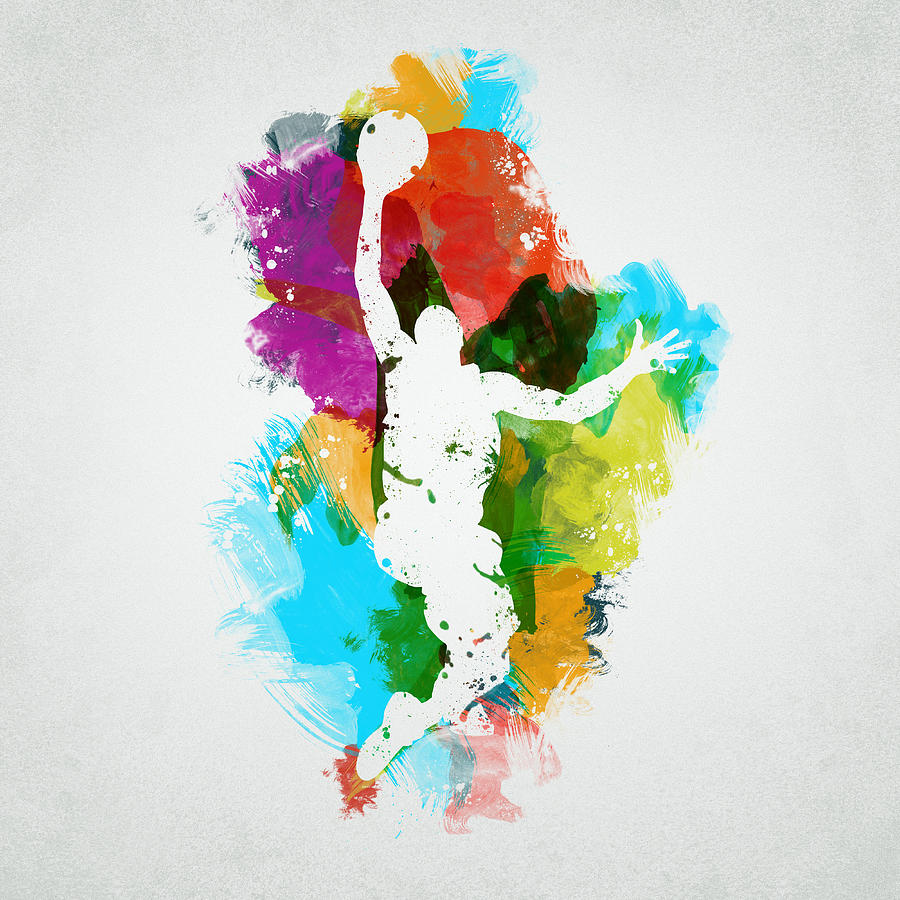The image features a dynamic, white silhouette of a basketball player mid-jump, with a seemingly upward gaze. The figure's right arm is extended upward clutching a basketball, while the left arm is stretched outward. The player's legs dangle as though captured in mid-air, the right knee slightly bent and higher than the left. Surrounding the white silhouette is a vibrant, abstract explosion of rainbow colors—reds, greens, blues, purples, oranges, and yellows—splashed like paint in broad, splotchy strokes that evoke a sense of energy and motion. The backdrop is a subtle light gray, providing a muted contrast that emphasizes the colorful, swirling background and stark white figure, lending the piece a sense of depth and dramatic focus.